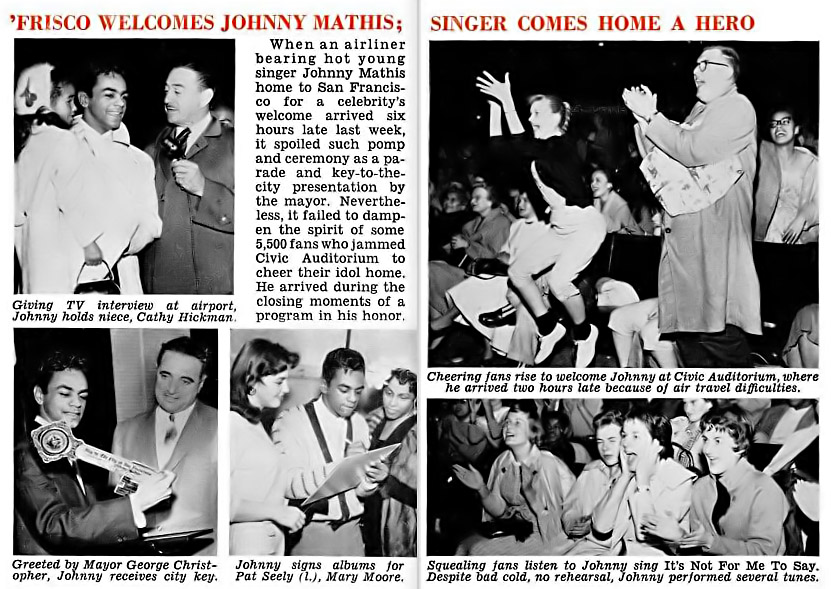The image is a scan of a magazine spread featuring text and several black and white photographs chronicling Johnny Mathis's delayed but spirited homecoming to San Francisco. At the top, the red heading reads, "Frisco welcomes Johnny Mathis." The accompanying article details how an airliner carrying the young singer arrived six hours late, disrupting planned celebrations like a parade and a key to the city presentation by the mayor. Despite this setback, 5,500 enthusiastic fans packed the Civic Auditorium to welcome Mathis during the concluding moments of an event held in his honor.

On the left page, three photos capture the scene: one shows Mathis giving a TV interview at the airport while holding his niece, Kathy Hickman; another depicts Mayor George Christopher presenting Johnny with the city key; and the final one shows Mathis signing albums for fans Pat Seely and Mary Moore. The right page continues with two more photos: one of cheering fans at the Civic Auditorium reacting to his late arrival, and another of the "squealing fans" as Mathis performs the song "It's Not For Me To Say," despite having a bad cold and no rehearsal. The collective joy and excitement of the fans underscore Mathis's heroic homecoming.